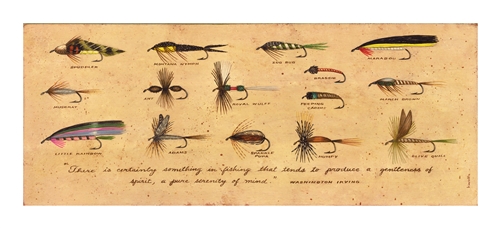The image depicts an array of meticulously illustrated fly fishing flies against a horizontally rectangular tan background, resembling an old, yellowed piece of paper. These flies are organized into three distinct rows: the top row features four flies, the middle row showcases five (with the second from the right displaying an additional fly above it, making it appear as if there are two), and the bottom row contains another five flies. These intricate flies, designed to mimic various insects like beetles, dragonflies, and mosquitoes, each sport fishhooks adorned with wings, legs, or fish-like features, and are rendered in multiple bright colors. Beneath each fly, there's a piece of handwritten black cursive text, likely naming or describing each fly, though it is too small to decipher clearly. At the bottom of the image, there's a handwritten inscription that reads, "there is certainly something in fishing that tends to produce a gentleness of spirit, a pure serenity of mind."